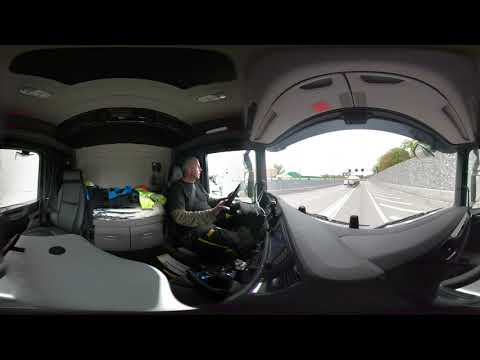The photograph is a panoramic color image with a fisheye filter applied, capturing a detailed interior and exterior view from inside a large vehicle, such as an RV or a big rig truck. The image is in landscape orientation and features a horizontal black strip across the top and bottom of the photograph, reminiscent of a cinematic frame. 

The left side of the image reveals an interior cabin scene, showcasing the dashboard and seating area. The dashboard is a blend of black and tan hues, while the ceiling is a light tan, likely leather or leather-like material. The seats are gray, and there is a tan shelving unit or console between them. A middle-aged white adult man, estimated to be around 50 years old, is at the helm. He's dressed in a black shirt with camouflaged green and tan sleeves and dark pants. The man is looking out through the driver’s side window, focused on the road ahead.

On the right side, the photograph provides a view through the windshield, presenting the traffic and environment outside. The scene includes a large semi-truck in the left lane, suggesting that the focal vehicle is in the right lane of a two-lane road. The road is black asphalt with white lane markings, flanked by a tan and black brick wall to the right. A few green trees are visible against the white sky background, adding a touch of nature to the otherwise urban landscape. The windshield wipers are visible at the bottom of the expansive windshield.

The photo style leans towards photographic representationalism, illustrating the scene with clarity and realism, enhanced by the panoramic and fisheye filters that provide a comprehensive, almost 360-degree view of both the vehicle's interior and the road outside.